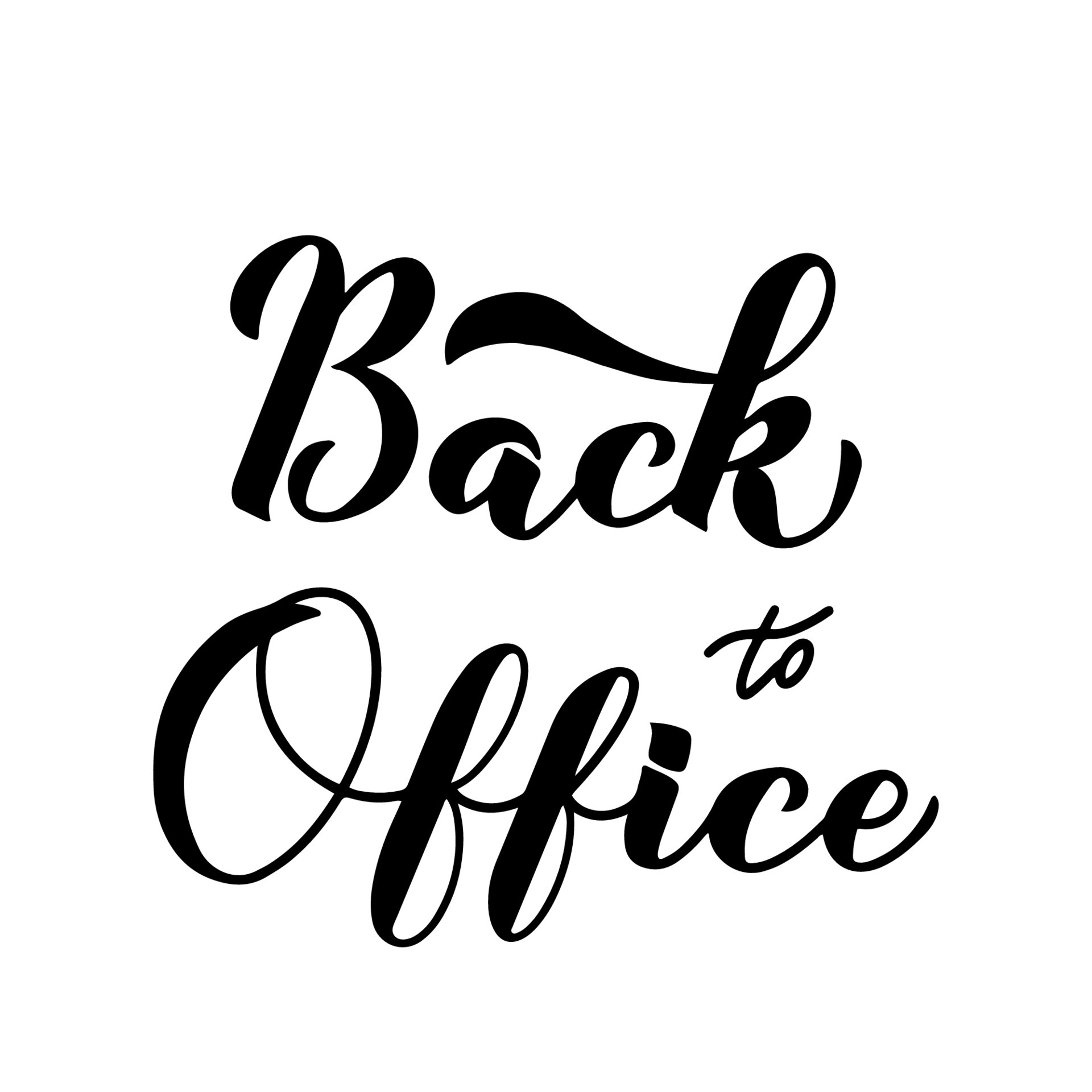The image presents a simple yet elegantly designed text on a plain white background. In bold black script, the prominent cursive font reads "Back to Office." Notably, the capital "B" and "O" stand out, with the letter "B" featuring a small embellishment that curves towards its center. Additionally, the "K" has a stylish ribbon-like embellishment that swoops back towards the "B." The word "to" is significantly smaller and positioned towards the right between "Back" and "Office." The overall design is minimalist, with no other elements present, emphasizing the sophisticated and straightforward message.